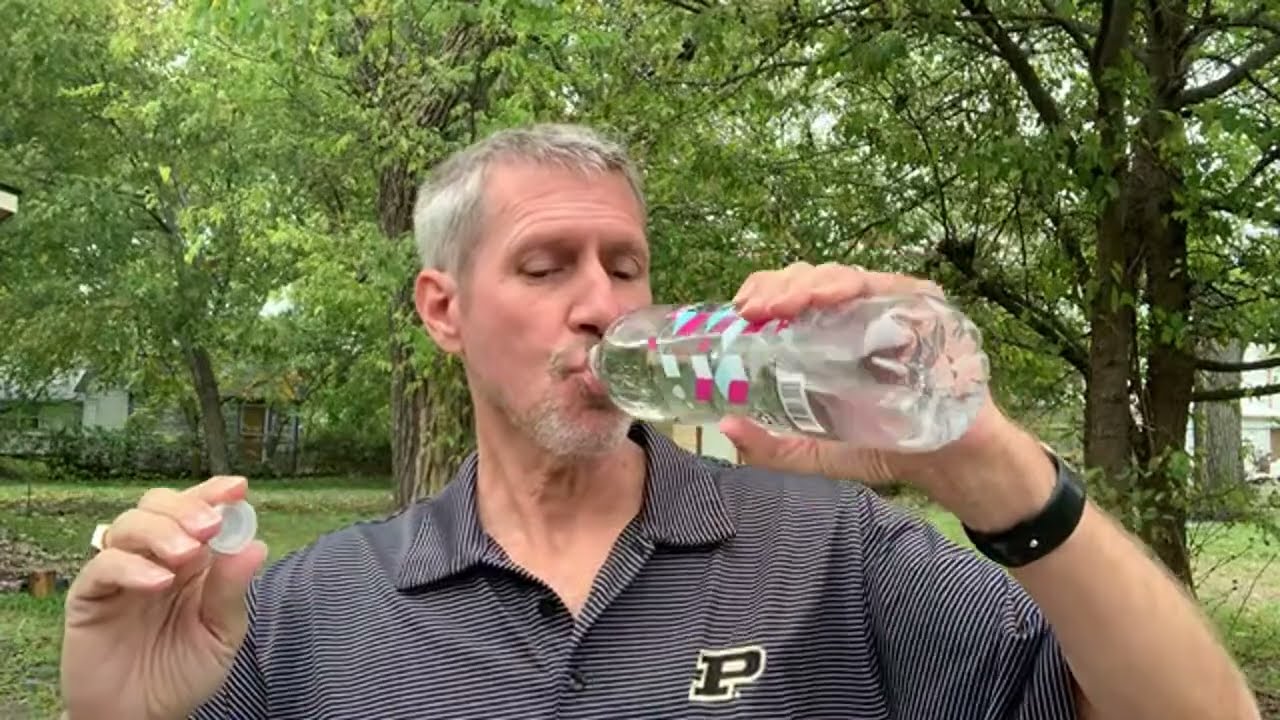The color photograph in landscape orientation captures a close-up view of a man outdoors in what appears to be a lush backyard or park setting with multiple mature trees. The man, who has prematurely white, short hair and a youthful face, is wearing a gray and white thin-striped polo shirt featuring a large green letter "P" with a white background on the left breast. He holds a nearly full plastic water bottle in his left hand, from which he is currently drinking, casting his downward-gazing eyes in a focused manner. His right hand holds the bottle cap, and on this hand, he wears a gold ring on his ring finger. Additionally, a black banded wristwatch or Fitbit adorns his left wrist. The background reveals a serene, verdant environment with tall trees extending their leaves overhead, and hints of a building behind a fenced area, adding to the tranquil suburban ambiance.